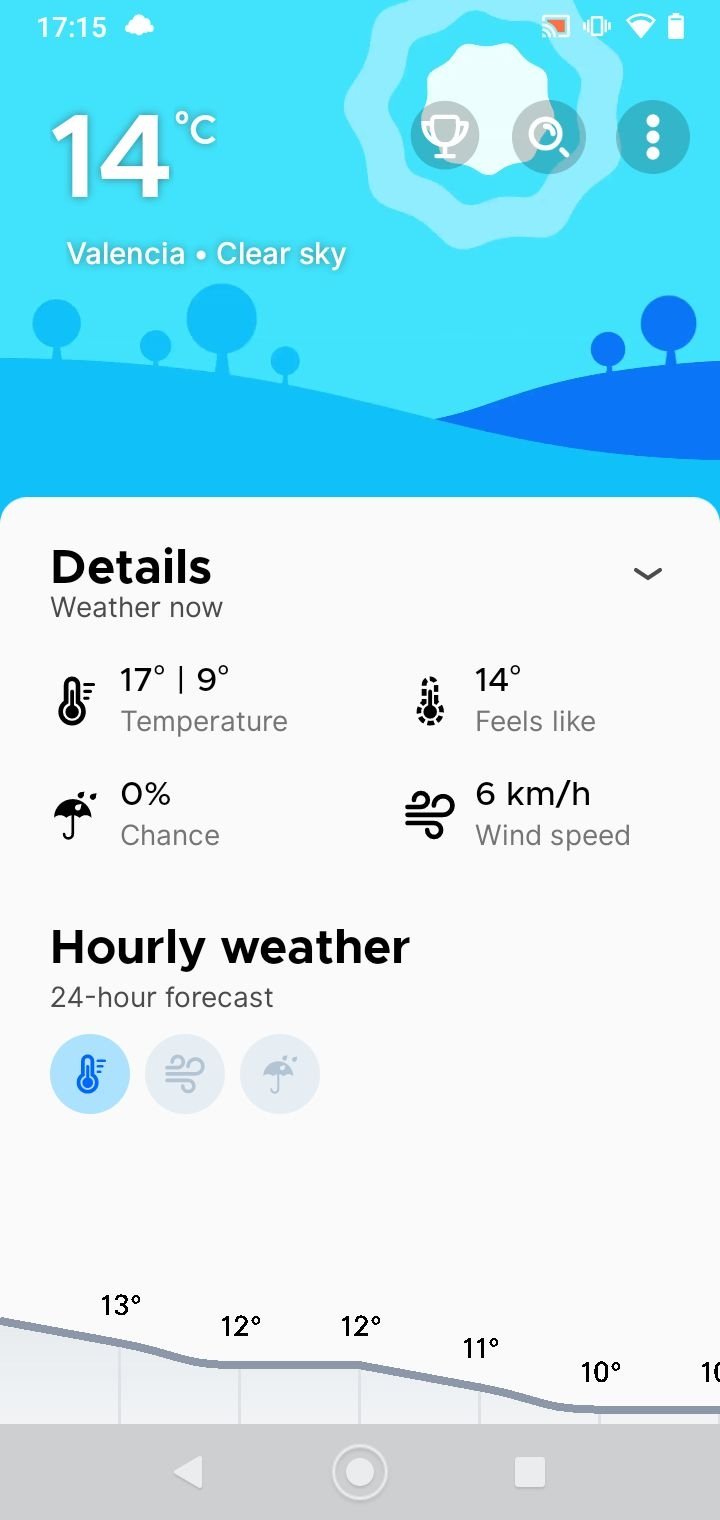The image showcases a detailed weather display on a piece of equipment. The vibrant blue background, transitioning from a deep to a sky blue, sets the tone for the weather information. Situated at the top right of the display are graphics depicting a sunny day with rolling hills and tree icons, reinforcing the serene weather theme.

The main weather data highlighted includes a current temperature of 14 degrees Celsius in Valencia, under clear skies. Additional details are provided below the main temperature: the day's high is expected to reach 17 degrees Celsius, with lows of 9 degrees Celsius, and a "feels like" temperature of 14 degrees Celsius. There's a 0% chance of rain, with a wind speed of 6 kilometers per hour.

The display also includes an hourly weather forecast for the next 24 hours and a graph illustrating the expected precipitation levels.